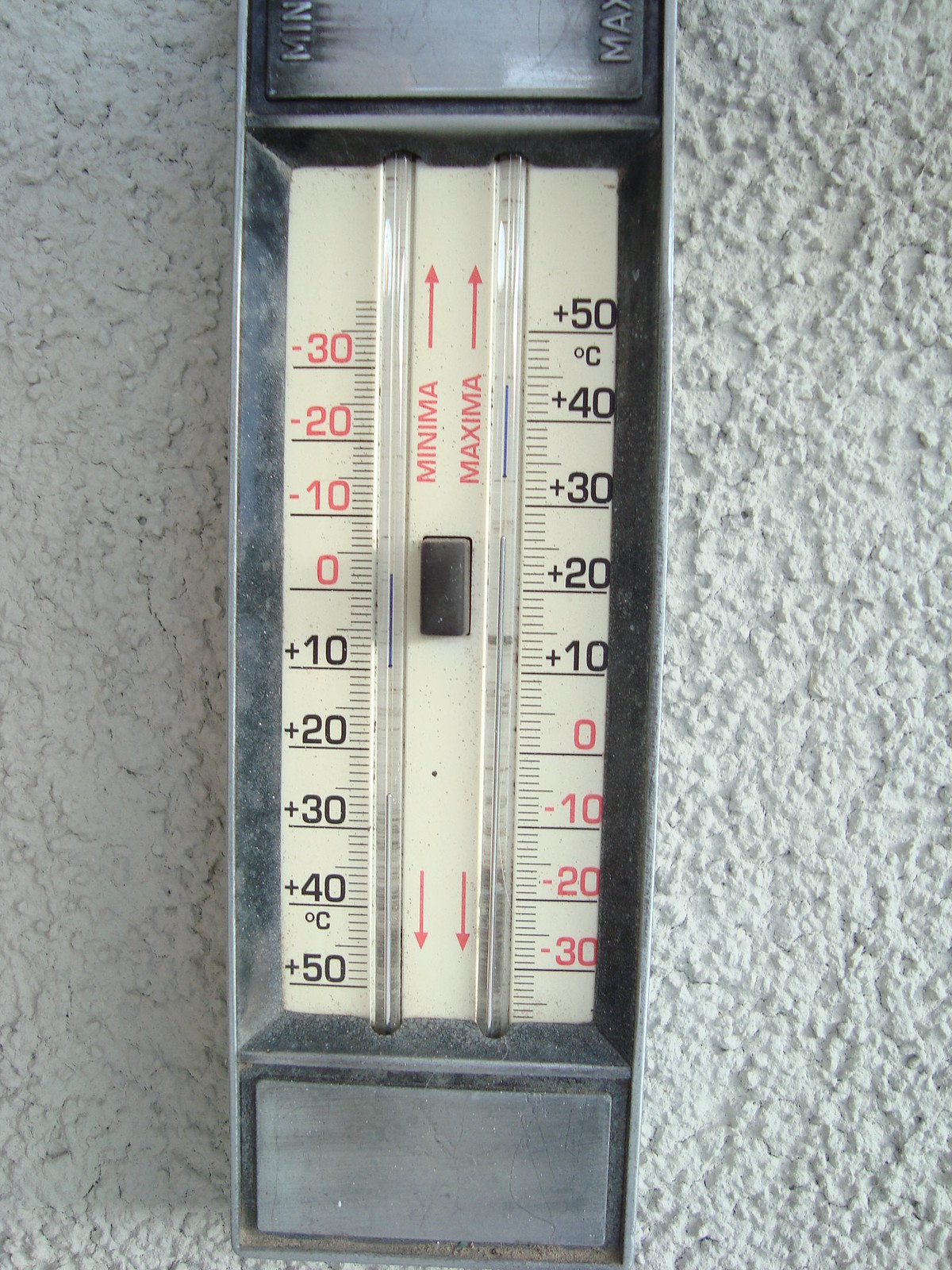The image is a realistic vertical photograph featuring a prominently displayed thermometer against a textured white wall, possibly stucco with a popcorn-like finish. The thermometer itself has a frame that appears to be made of stainless steel, with metallic silver-gray edges running vertically along both sides. The bottom and top of the thermometer are capped with horizontal metal bars, potentially serving as reservoirs for the liquid inside.

The center of the thermometer houses two parallel glass tubes, and the background is a light beige color, enhancing readability. A small black button is located centrally between the two tubes.

In the upper middle part of the thermometer, red text labels "minima" with an upward-pointing arrow to the left tube and "maxima" with an upward-pointing arrow to the right tube. Below these labels, at the lower middle section, are arrows pointing downwards.

On the left side of the thermometer, aligned vertically next to the glass tube, red text marks the temperature in descending order: 0, -10, -20, and -30 degrees Celsius. Below this, in black text, is an ascending temperature scale: +10, +20, +30, +40, and +50 degrees Celsius.

On the right side, the temperature scale is mirrored in black text, starting from +10 to +50 degrees Celsius from the center upwards. Below the center, descending in red text, are markings for 0, -10, -20, and -30 degrees Celsius. The deliberate use of color and placement for the text ensures clear differentiation between positive and negative temperature readings.